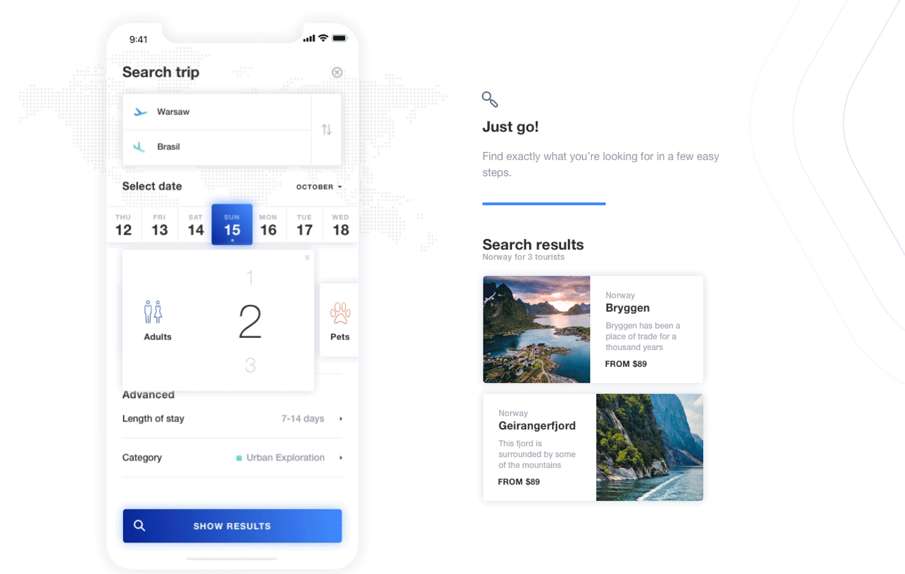The image showcases two distinct screens side by side. On the left, there is an iPhone screen featuring a visible notch, devoid of any bezels. The screen displays a travel search interface with the heading "Search Trip" at the top. The options presented include two destinations: Warsaw and Brazil. Beneath this, the user has selected specific details: travel dates spanning from December 12th to the 15th, a group size of two adults, a planned stay duration of 7 to 14 days, and the category specified as urban exploration. At the bottom, there is a prompt to "Show Results," implying an impending search for flight tickets, likely from Warsaw to Brazil, although it is not explicitly stated.

On the right, there is a simple rectangular image without any additional framing. It contains a motivational text encouraging users to "Find exactly what you're looking for" in "a few easy steps." Below this, the search results display places in Norway, featuring two scenic locations that appear enticing. This section seems to serve a different purpose or highlight a separate functionality compared to the left screen.